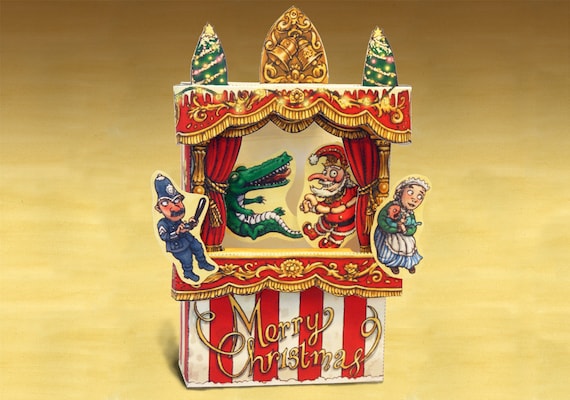The image depicts an intricate diorama designed to resemble a puppet show or miniature theater. The backdrop, reminiscent of a wooden surface with its yellowish-tan hue, enhances the nostalgic ambiance of the scene. Dominating the forefront is a vibrant red and gold structure adorned with lavish decorations and a fringed curtain that wraps around the scene, held back by ropes. "Merry Christmas" is elegantly scrawled in gold cursive at the bottom, set against a striking backdrop of alternating red and white stripes.

On the left side of the stage stands a classic United Kingdom policeman figurine, known as a "Bobby," in a tall blue hat, blue uniform, and holding a truncheon. Opposite him, a woman in a long blue dress with a white ruffled hem cradles a baby, her gray hair styled neatly. Center stage features a playful cast of characters: a green crocodile with a red tongue, white teeth, and a white belly, and a lively Santa Claus figure dressed in a red hat with a white pom-pom, a red shirt, red pants, elf-like shoes, and a tan belt. Santa's distinctively exaggerated long nose and white beard add a whimsical touch. Atop the scene, two small Christmas trees frame the festive display, completing this charming and detailed holiday diorama.